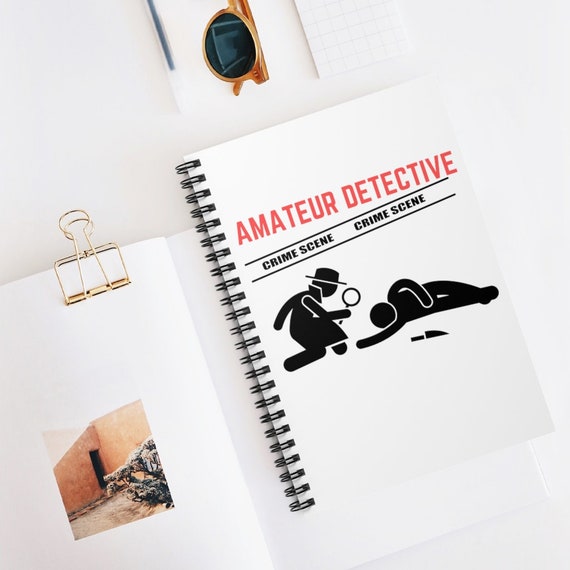This image shows a top-down view of a pristine white desk or table. Central to the image is a squarely framed, diagonally tilted spiral notebook with a black spiral binding. The notebook's white cover prominently features the words "Amateur Detective" in bold red letters at the top. Beneath that, positioned like police crime scene tape, "Crime Scene" is repeated within black-and-white striped borders. Below this tape, there are two black stick-figure silhouettes: one depicts a detective wearing a hat and coat, holding a magnifying glass and inspecting a fallen body with a knife nearby. Resting above the main notebook is a pair of brown sunglasses, and partially tucked behind it, a second white book held open by a gold page clip. This second book reveals an image of a tan, rust-colored building corner with a black doorway, green shrubbery, and a dirt ground, adding depth and intrigue to the detective theme of the setup.